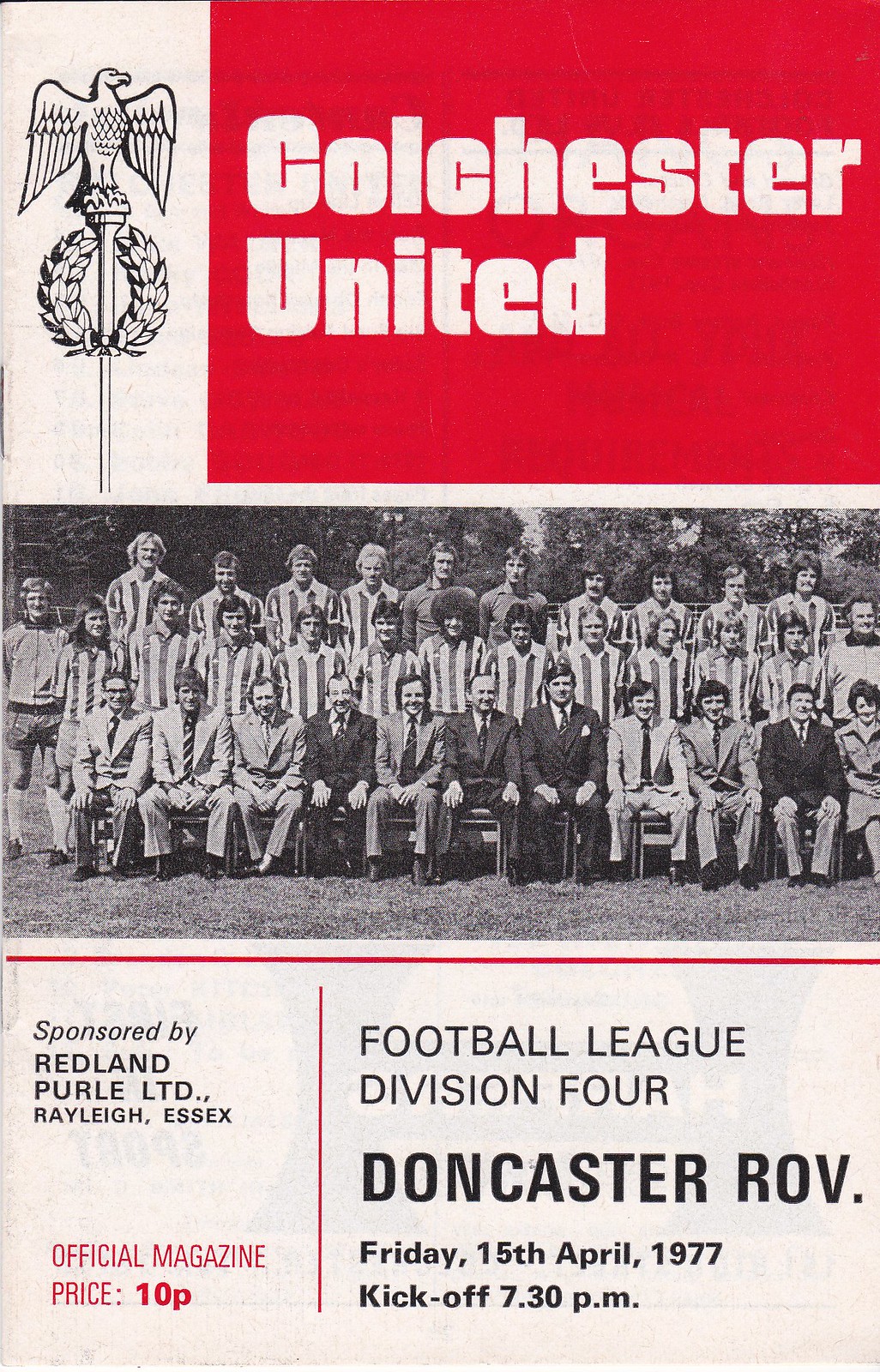The image is the cover of a vintage soccer program for Colchester United, dating back to April 15, 1977, which has aged over time with noticeable browning and blemishes on the paper. Dominating the top third of the page, a red rectangle is prominently placed on the right, emblazoned with the team name "Colchester United" in bold white letters. To the left of this is a striking black and white illustration of an eagle with outspread wings perched on a pole, accompanied by ornamental details below it.

Beneath the illustration, a black and white team photograph captures the entire squad. The team officials, dressed in suits, are seated in the front row, showcasing a range of ages from older men to those in their 20s and 30s. Behind them, the players stand in two rows, sporting striped jerseys typical of the era. Below the photograph, text indicates the sponsorship by Redland Pearl Limited, Raleigh, Essex, and in red letters, it states "Official Magazine, price 10 pence". Further down, on the right side, additional text provides details about the football match: "Football League Division IV, Doncaster ROV," and specifies the event's date and time as Friday, 15th April 1977, with a kickoff at 7:30 p.m.